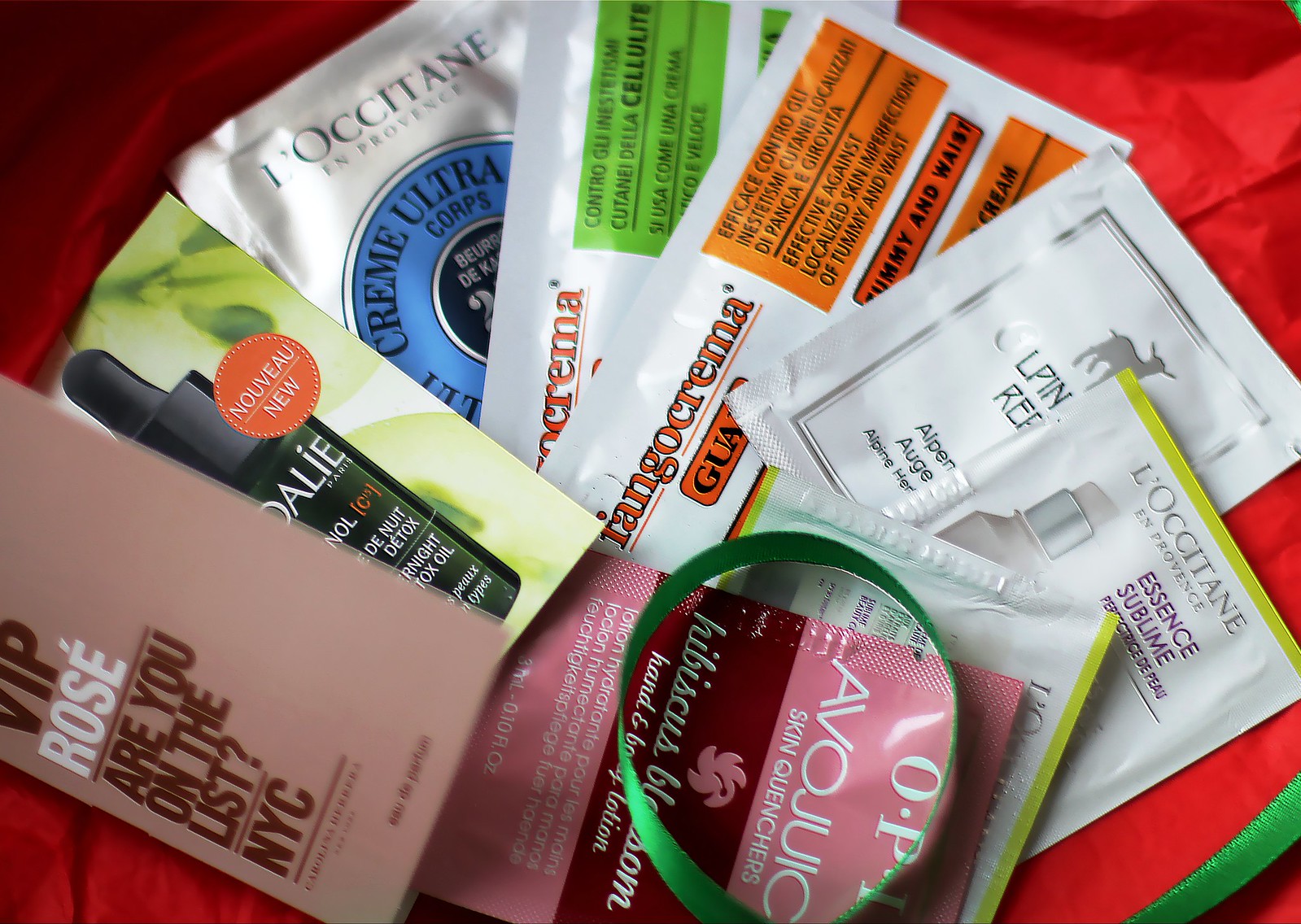This color photograph presents a close-up view of several small foil packets, containing a variety of cosmetic samples, artfully arranged against a striking backdrop of vibrant red cloth. The lower right-hand corner of the cloth features an intricate green embroidery border, adding a touch of elegance to the composition. On the left side of the image, part of a brochure is visible, characterized by a dusty pink color. The brochure prominently displays the text "VIP Rose: Are you on the list?" followed by "NYC" for New York City.

Among the array of sampler packets, one stands out with a discernible image of a black cosmetic bottle adorned with white lettering. This packet also features an orange seal labeled "nouveau," indicating it as a new product. Next to it, another packet, although slightly blurry, displays a turquoise blue circle with the words "cream ultra" inscribed within it. The fine print across most of the packets is too small to read, but their varied colors and designs suggest a diverse selection of cosmetic products.